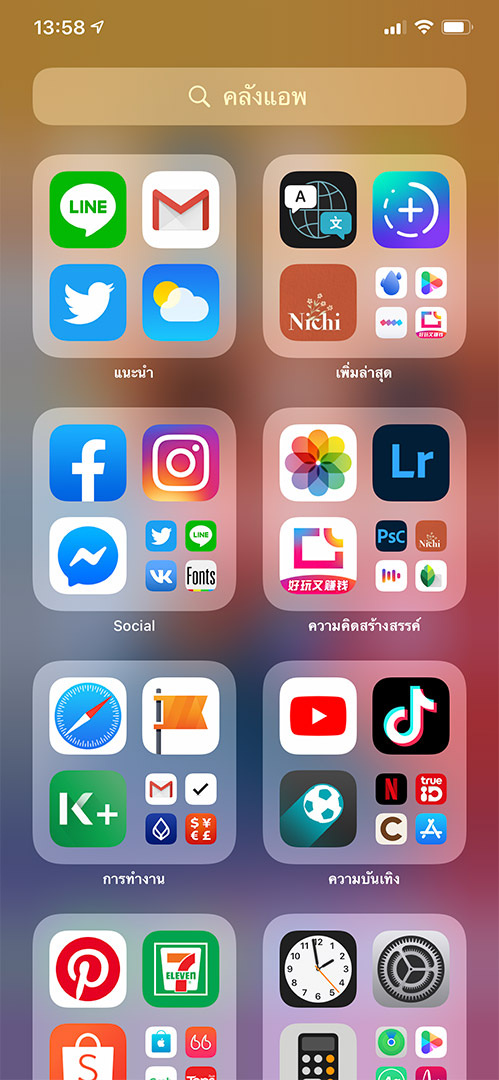This is an image capturing a smartphone home screen with a tan-colored background. At the top, there is a search bar displaying white text in a foreign language. The time on the phone reads 13:58, located at the upper right corner, where the battery indicator shows a mostly full charge, and the connection status appears to be strong. The home screen is densely populated with possibly over 50 applications. Notable among these apps are Safari, Facebook, Instagram, Twitter, a clock indicating almost two o'clock, 7-Eleven, Pinterest, a music app, and a font app.